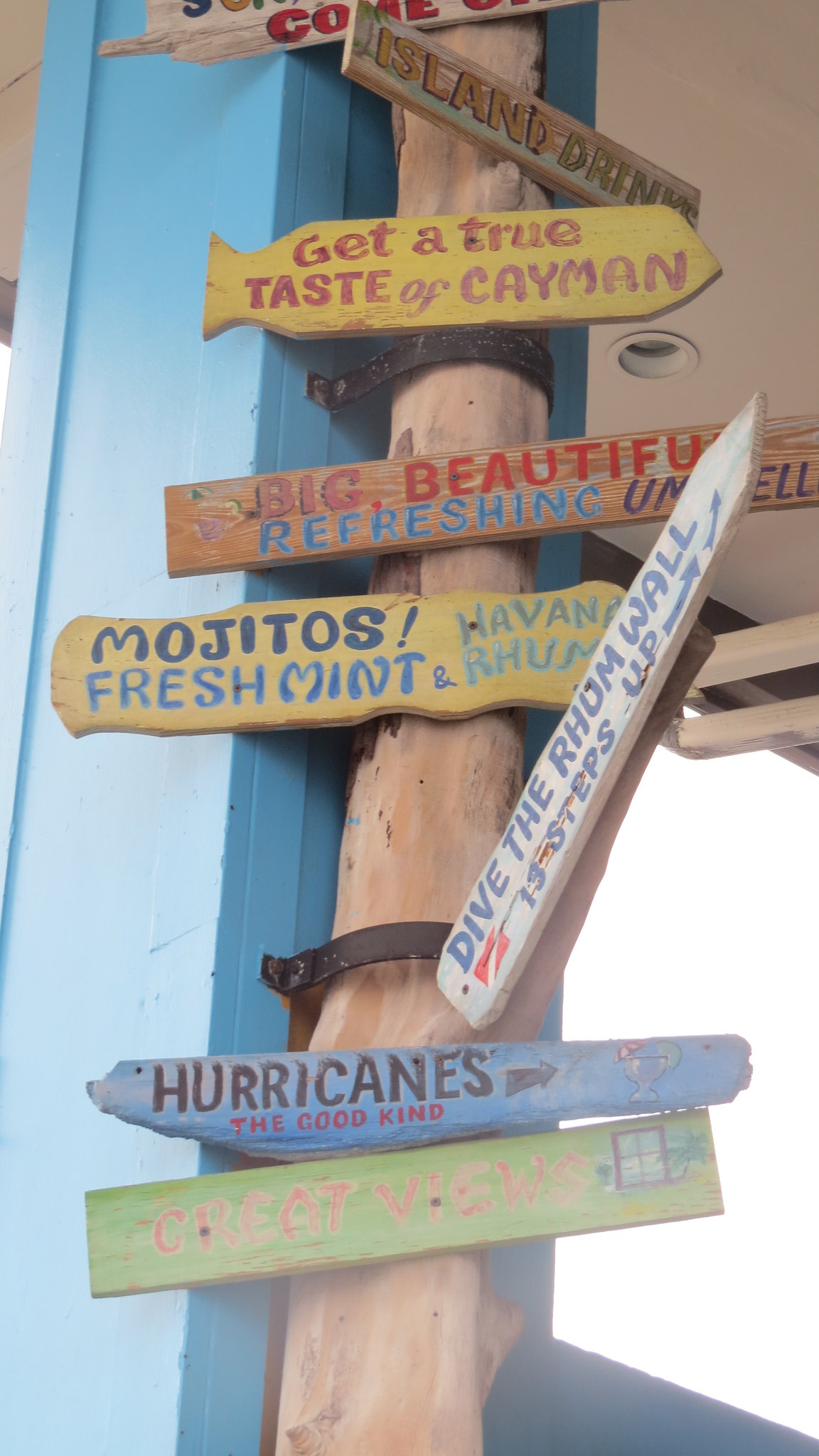The photograph showcases a tall, whimsical signpost made from a tree trunk-like blue post with various colorful signs arranged at different levels, pointing in multiple directions. The vibrant signs are either pointing left, right, or upward and feature catchy and inviting messages suggestive of a vacation hotspot. At the top, a sign reads, "Come Something," followed by "Island Drinks," evoking thoughts of a tropical paradise. Further down, a yellow, fish-shaped sign with the message "Get a True Taste of Cayman" points to the right, suggesting a local fish restaurant. Another sign reads, "Big Beautiful Refreshing Un..." with incomplete text, while "Mojitos Fresh Mint Havana Rum" promises a refreshing drink experience. The sign "Dive the Run Wall, 13 Steps Up" hints at a diving attraction nearby. One of the lower signs, in blue, points to the left and says, "Hurricanes, The Good Kind," likely indicating a bar. The overall impression is one of a lively and inviting area, with each sign adding to the colorful, light-hearted atmosphere of the locale.